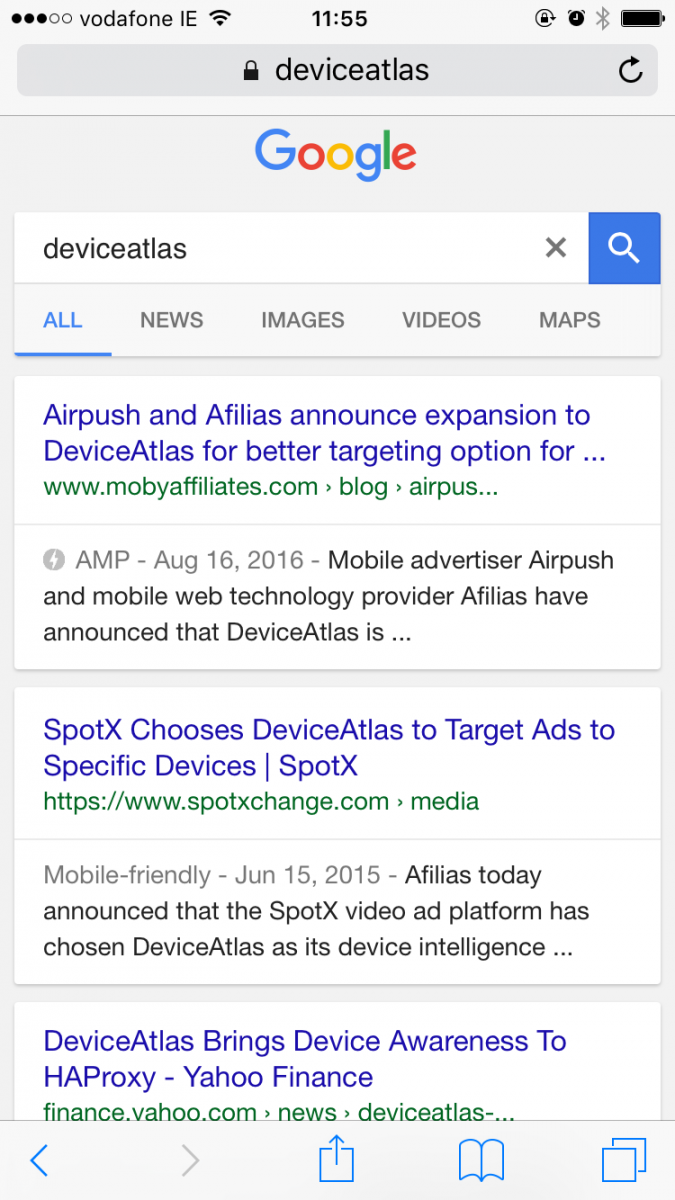This image is a screenshot of a Google search results page on a Vodafone device, captured at 11:55 AM. The top search bar displays the query "DEVICEATLAS," with the Google logo preceding the search box. Below the search box are the standard categories: "All," "News," "Images," "Videos," and "Maps."

The first search result, highlighted in blue, reads: "AirPush and Afilias announce expansion to DeviceAtlas for better targeting options..." with a link to www.mobileaffiliates.com. Additional details under this heading include the words "blog" and "AirPush."

The second search result, dated August 16, 2016, is from Mobile Advisor and reads: "AirPush and mobile web technology provider Afilias have announced that DeviceAtlas is..."

The third search result, also in bold blue, is titled: "SpotX chooses DeviceAtlas to target ads to specific devices, SpotX." The corresponding website is https://www.spotexchange.com, listed under the text "era media" in green. The summary notes: "Afilias today announced that SpotX video ad platform has chosen DeviceAtlas as its device intelligence..."

The final search result in bold blue states: "DeviceAtlas brings device awareness to HAProxy - Yahoo Finance." The related website, finance.yahoo.com, is listed under the heading "era news, era DeviceAtlas."

Each search result snippet provides a snapshot of how DeviceAtlas is utilized in various technological and marketing contexts, highlighting partnerships and applications in targeting and device intelligence.